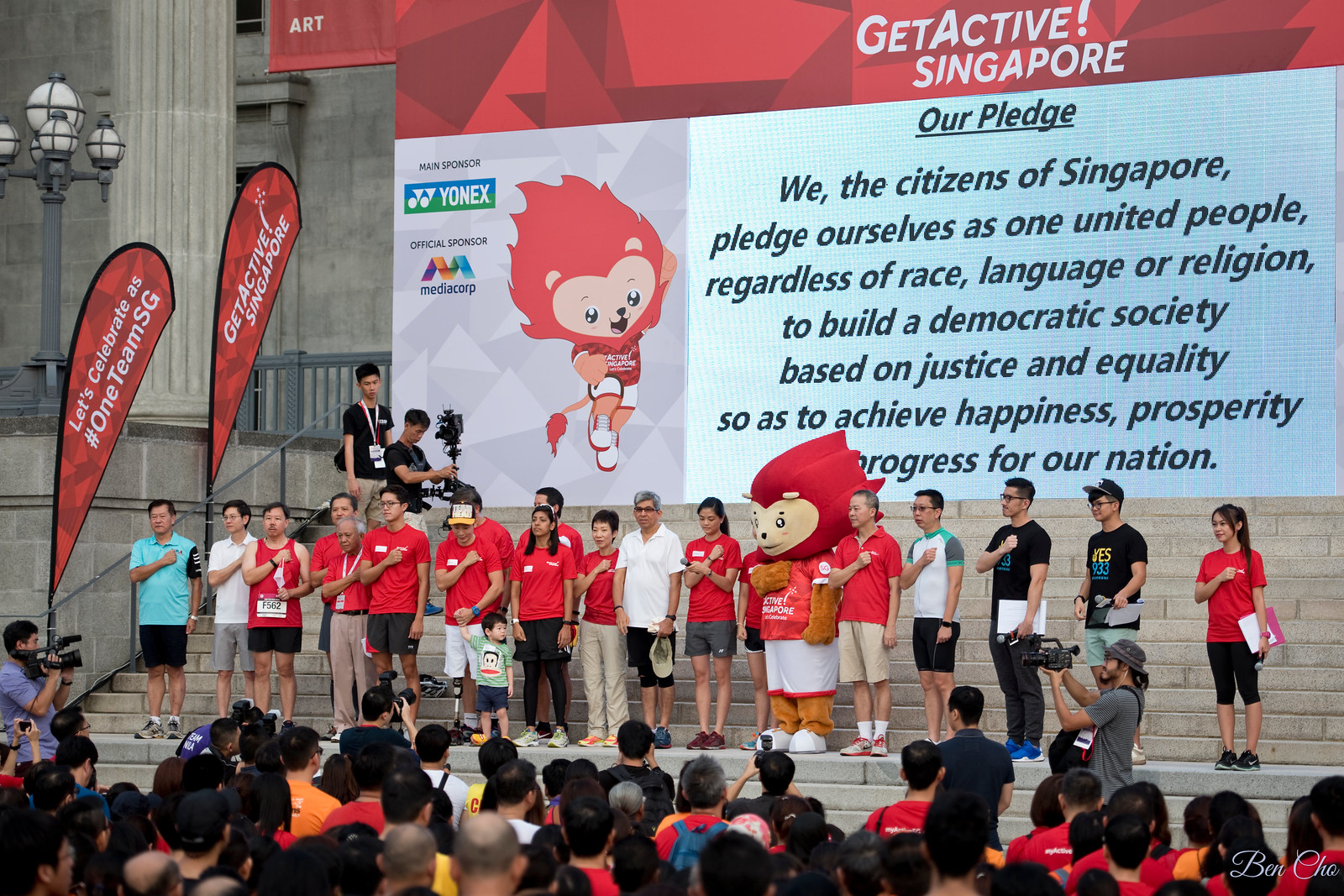In a bustling public square in Singapore, a diverse group of individuals stands in a line atop the cement stairs of a grand grey marble building, participating in an event organized to promote fitness and unity under the banner "Get Active Singapore." Most of the participants are uniformly dressed in red shirts, embodying the spirit of the event. Among them is a lively lion mascot, dressed in sports trunks and a jersey, with a big red mane, a cartoonish cute face, and big white shoes, adding an element of fun to the proceedings. Behind the group, a large banner prominently displays the Singapore Pledge: "We, the citizens of Singapore, pledge ourselves as one united people regardless of race, language, or religion to build a democratic society based on justice and equality so as to achieve happiness, prosperity, and progress for our nation." In front of the stairs, a crowd of spectators gathers, some with cameras in hand, capturing the moment. On the left side of the scene, a camera crew dressed in black shirts can be seen documenting the event, which highlights a collective commitment to fitness and national unity.